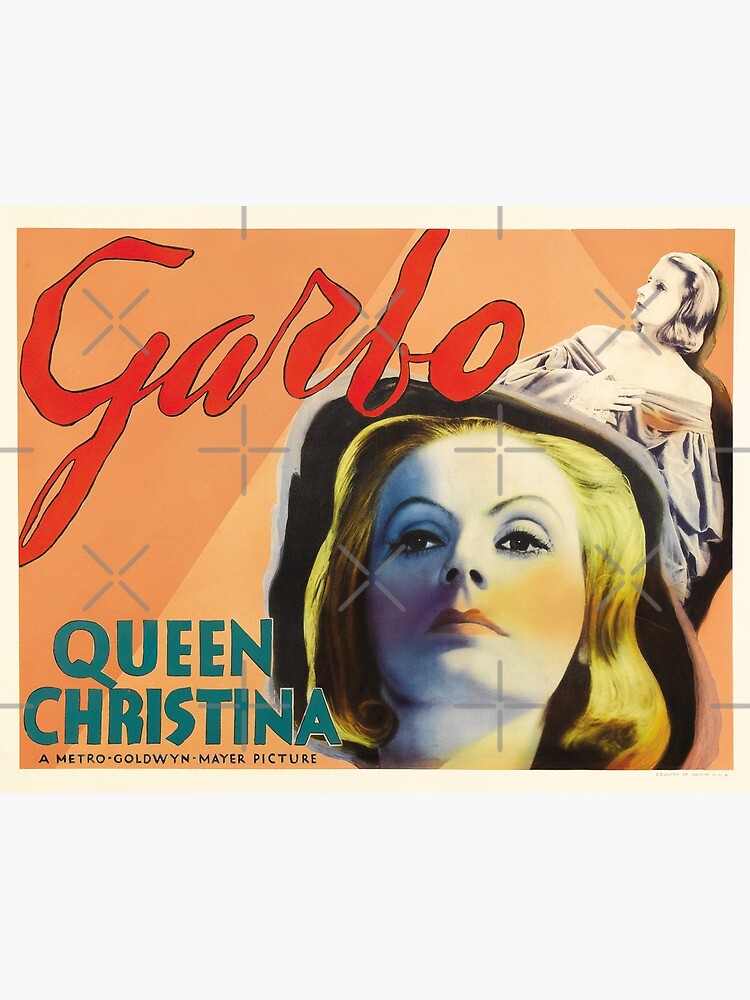The image is an advertisement poster for the movie "Queen Christina," prominently featuring actress Greta Garbo. The rectangular poster background transitions through various shades of orange, with a lighter orange streak running through the right side. At the top left, "Garbo" is written in bold red cursive, dominating a significant portion of the space. Below it, in green bold capital letters, is the movie title "Queen Christina," followed by "a Metro-Goldwyn-Mayer picture" in a smaller blue font.

In the foreground, there's a vibrant colorized image of Greta Garbo with blonde hair, pale skin, and prominent red blush and lips, looking upwards and to the left. This image occupies the bottom right corner and extends midway up the poster. Behind it, another, more subdued black-and-white image of Garbo is visible, portraying her from the bust up, gazing in the same direction and clutching her dress, adding depth and a reflective motif to the design. No other individuals are present in the artwork.